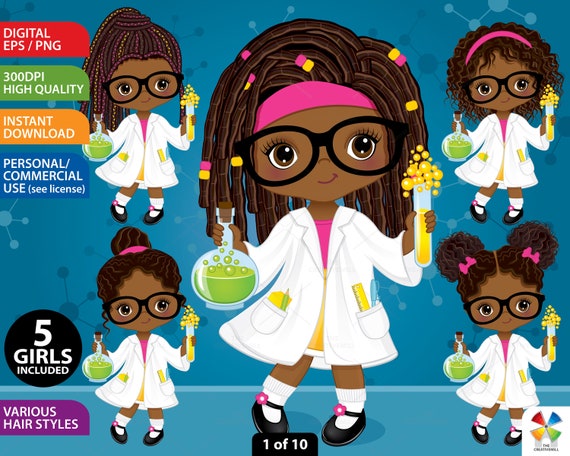The image is an advertisement, likely a screen grab, with a blue background featuring chemical atom structures and models. In the center is a larger cartoon depiction of a young Black girl with braided hair, an ornament in her hair, black glasses, and a pink headband. She wears a pink shirt under a white lab coat, with various items in its pockets. She holds a beaker with green liquid in one hand and a test tube with yellow liquid in the other, both of which are bubbling. Surrounding her are four smaller, similar characters, each with different hairstyles but also wearing white lab coats and holding beakers and test tubes. The image includes text in various colors and backgrounds on the left, such as "Digital EPS/PNG," "300 dpi, high quality," "Instant Download," and "Personal/Commercial Use (C License)." A black circle with white lettering states "Five Girls Included," and a purple background with white text highlights "Various Hairstyles." At the bottom center, it says "One of Ten" on a black background, and the lower right features a colorful pinwheel resembling a windmill.